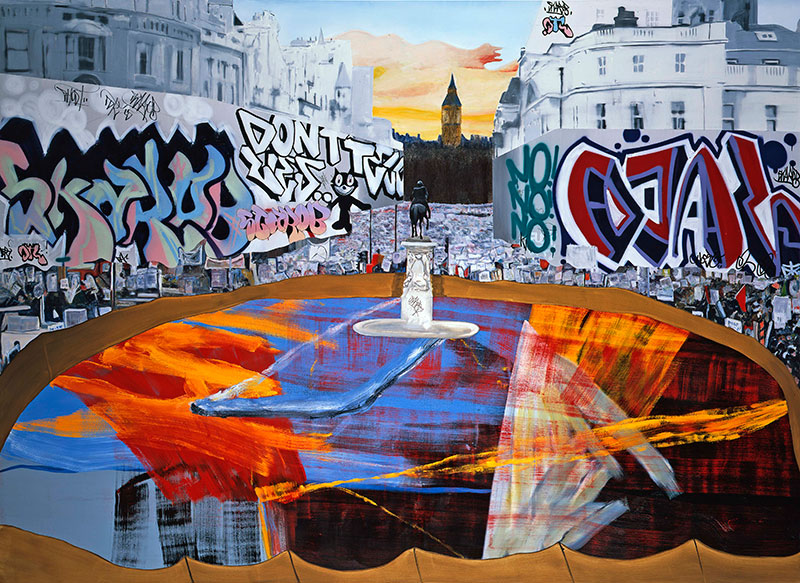The image is a highly detailed and vibrant artwork that merges elements of painting and collage. In the foreground, there's a prominent brown border that resembles a fountain, filled with vivid water-colored streaks in red, orange, blue, brown, and grey. Central to the image is a concrete pedestal, atop which stands a bronze statue of a person on a horse. Surrounding the pedestal are towering white buildings, their walls extensively covered in graffiti, including the words "don't" and "no" repeated multiple times, along with figures like Felix the Cat. Above, the sky is a striking mix of amber, red, and yellow sunset hues blending into blue. In the far background rises a tall building, reminiscent of architectural landmarks from Paris or England, possibly resembling the Big Ben Tower. Amidst the urban scene, there's a crowd of people, possibly holding signs, adding to the bustling and layered atmosphere of the setting.